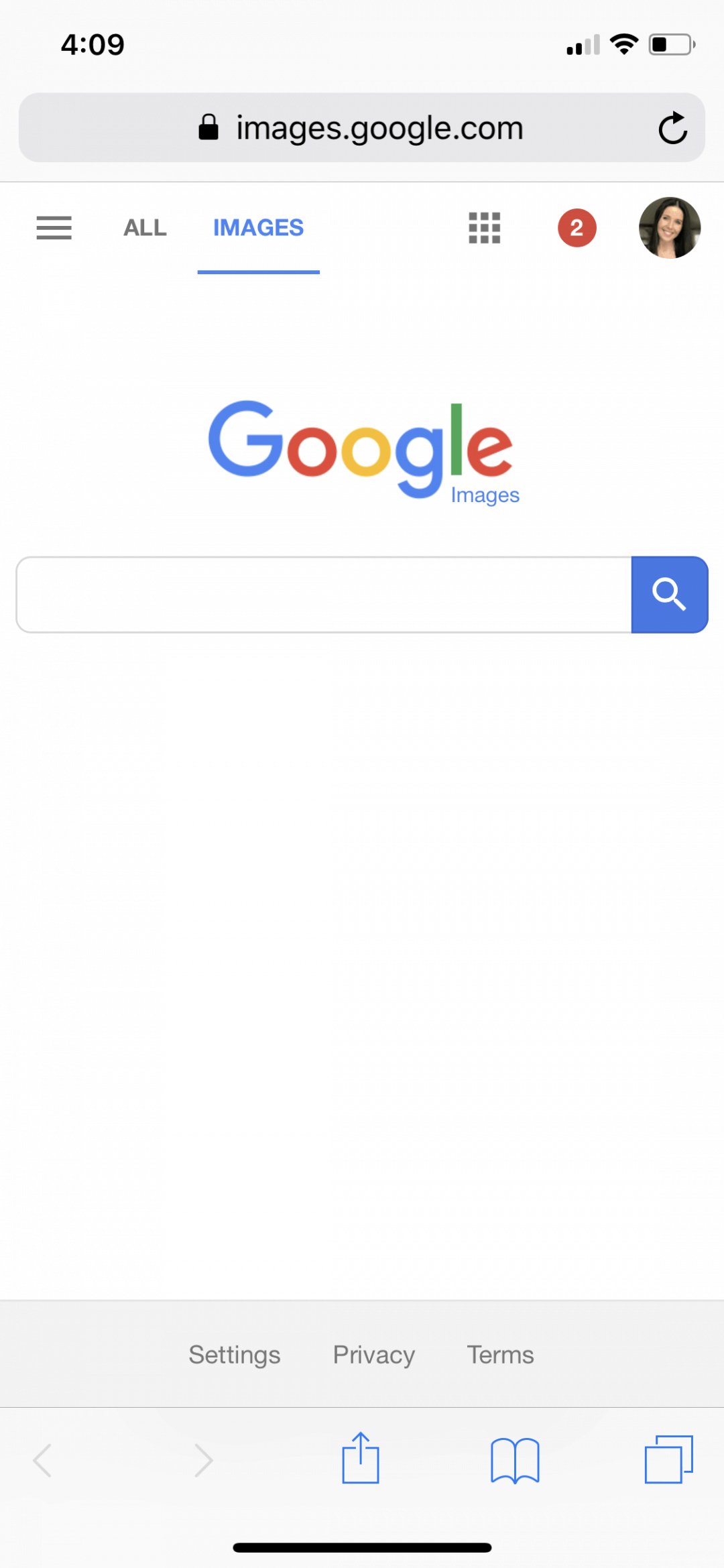A detailed screenshot from a mobile device displaying Google Images page. At the top of the screen, the time is 4:09. The status bar shows a coverage icon, a Wi-Fi icon, and a nearly depleted battery icon. Just beneath, a gray search bar is present with a black padlock icon and the text "images.google.com" in black. A circular refresh arrow pointing to the right is positioned at the far-right end of the bar. 

Below the search bar, the interface features several icons: three horizontal lines, an "All Images" tab currently selected, a grid icon made up of nine smaller squares, a red notification circle with the number 2 in white, and a circular profile photo of a young white woman with long, dark hair smiling while looking at the camera, her head slightly tilted to the right. 

The Google logo follows, colored traditionally with the first "G" in blue, the first "O" in red, the second "O" in yellow, the second "G" in blue, the "L" in green, and the "E" in red. Beneath the letters "L" and "E" is the word "images" in blue. 

Further down, there is another search bar with a blue section on its right end, featuring a white magnifying glass icon. At the very bottom of the screenshot, text links for "Settings," "Privacy," and "Terms" are displayed.